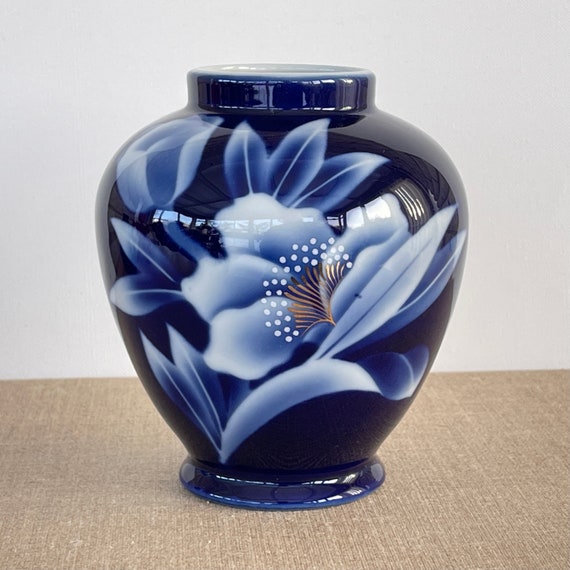The image features an exquisitely glossy, dark navy blue porcelain vase with an apple-like shape, tapering at the top and bottom with a subtle lip at its base. The vase displays a stunningly detailed floral pattern, featuring a large white flower with light blue leaves which include intricate veining. The flower has a copper-colored center with gold pollen and tiny white dots, providing a striking contrast to the dark background. The vase is placed on a brownish-creamy fabric or table, which adds a warm undertone to the scene. The high gloss finish of the vase reflects the surrounding room, including windows, adding depth and dimension to the picture. The background features a white, slightly grayish wall, enhancing the rich navy hue of the vase and making it the focal point of the image.